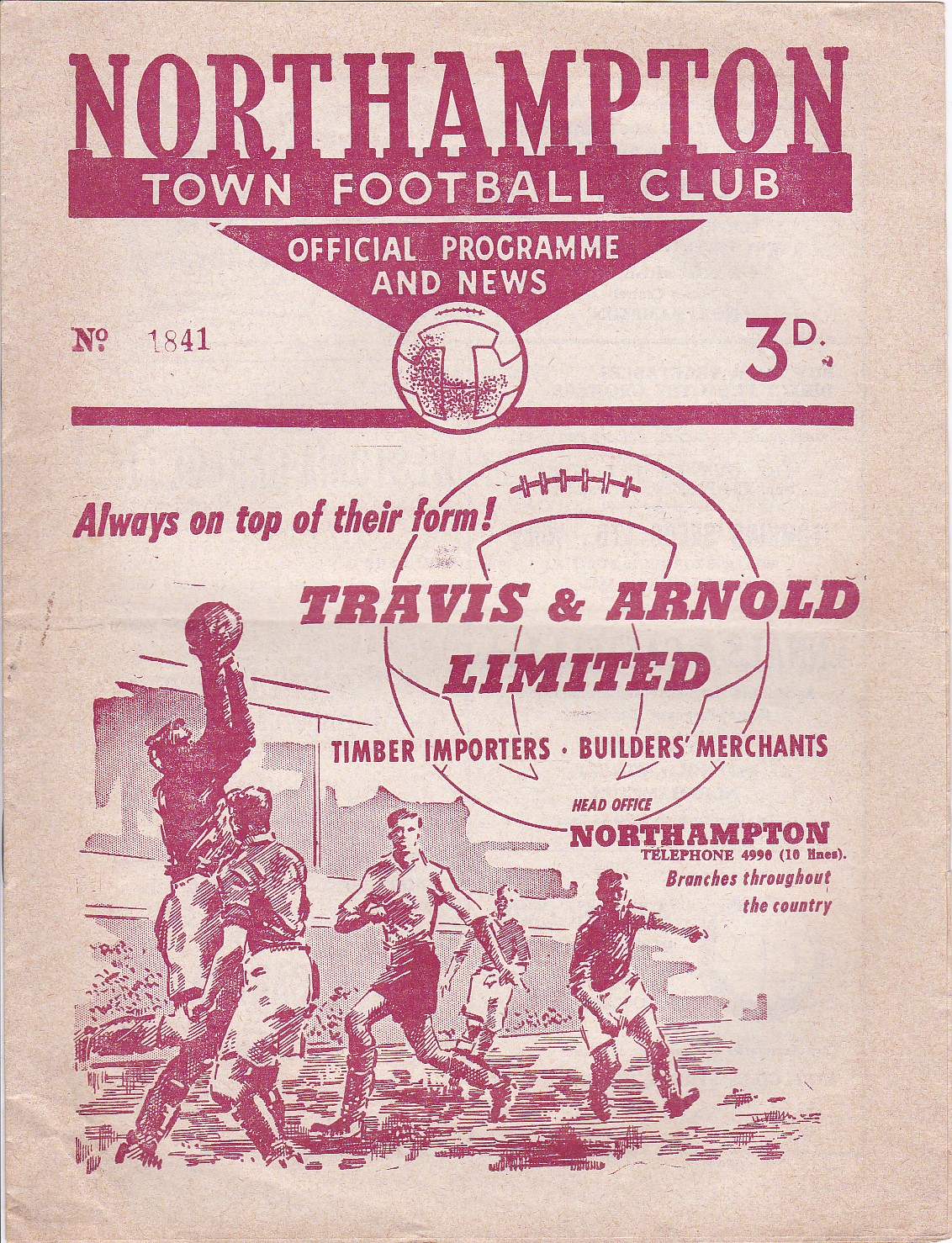A worn and vintage poster advert, possibly for a European soccer match, dominates the scene with its aged and discolored background, giving it a pale pinkish hue. Vibrant red text and limited color usage highlight its antiquated charm. At the top, it proudly announces "Northampton Town Football Club Official Program and News," with "NO 1841" featured to the left and "3D" to the right. A striking red line separates this header from the rest of the content. Below the line, an illustration of a dynamic soccer match draws the eye—players are caught mid-motion with one figure, likely a goalie, leaping up with the ball as other players rush toward him. Accentuating the energetic scene, the text beneath reads "Always on Top of Their Form." In the backdrop, a soccer ball subtly anchors the theme. Further down, in smaller print, the text advertises "Travis and Arnold Limited, Timber Importers, Builders, Merchants, Head Office: Northampton, Telephone 4996, Branches Throughout the Country."